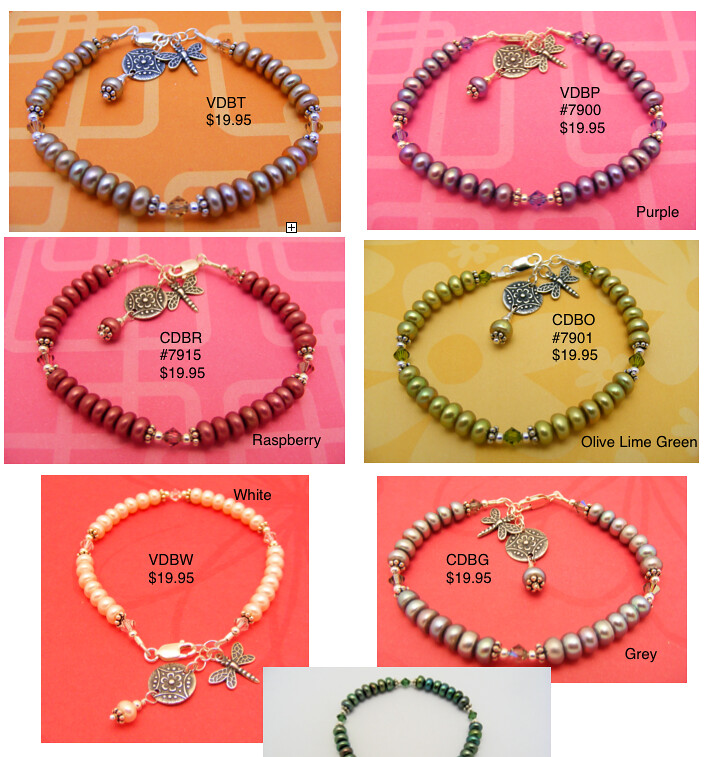This image appears to be a detailed catalog page featuring a variety of jewelry items. There are a total of seven bracelets displayed against various colored backgrounds, each priced at $19.95. 

In the upper left corner, there is a necklace with silver beads and an orange surface adorned with light patterns. It has a blue butterfly charm and a blue metal circle with a flower pattern from which silver beads hang. The item is labeled "VDBT $19.95."

Next to it on the upper right, set against a pink background, is another silver-beaded necklace tagged as "VDBP number 7900" with the same price of $19.95.

In the middle left section, against a light gray background, is a necklace with red beads, identified as "CDBR 17915 $19.95." Just below this, you’ll find a yellow-beaded necklace on a yellow background, marked "CDBO number 7901" also priced at $19.95.

Near the bottom left on a pink background is a necklace featuring white beads. This piece is labeled "VDBW $19.95." 

On the lower right, displayed against a pink backdrop, is a necklace with light gray beads, labeled "CDBG $19.95."

The overall presentation suggests a variety of beaded necklaces with unique charms such as a blue butterfly, a round metal piece with a flower pattern, and a dragonfly. The image clearly belongs to a catalog page, and no people are shown wearing the accessories.